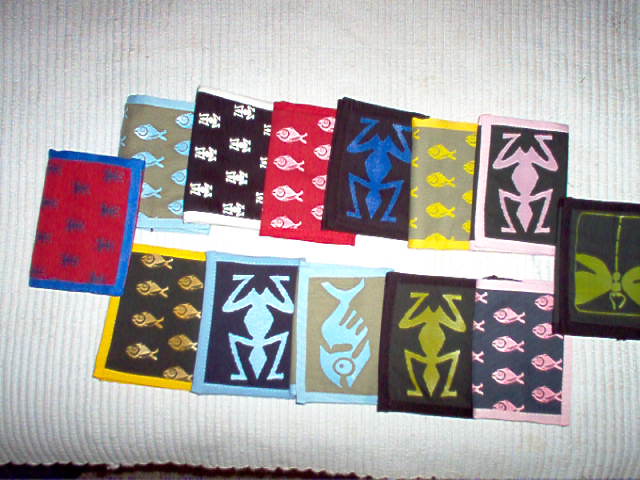The image, taken from a top-down perspective, depicts 14 colorful objects that resemble wallets arranged on a white, ribbed throw rug, possibly a quilted bedspread or a tablecloth. There are two rows of six wallets each, with one wallet on either side of the rows. Each object features unique and vibrant patterns, predominantly colorful fish and frogs, against dark backgrounds with contrasting light-colored trims.

Starting from the left, the wallet at the end is red with a blue trim and blueprint. In the first row, moving left to right: the first wallet has a yellow border, a black background, and a yellow fish design; the second shows a blue border, a black background, and what appears to be a frog viewed from above; the third, bordered in blue, has a light brown background with light blue fish; the fourth wallet features a black border, black background, and the same frog motif; the fifth has a pink border, black background, and numerous small pink fish; and the sixth wallet displays a light blue border with a brown background and blue fish.

Above these in the second row, again from left to right: a wallet with a white border, black background, and multiple white frogs; another with a red border and red background adorned with white fish; black-bordered with a black background and an upturned blue fish; yellow border with a green background showcasing yellow fish; and pink-bordered with a black background containing pink fish. Finally, lying at the rightmost end of the second row, a wallet features a gray background with a black trim and depicts a detailed green dragonfly design.

This visually rich collection is arrayed on a well-lit, possibly flash-assisted photograph, which brings out the intricate details and vivid colors against the contrasting white, ribbed surface.